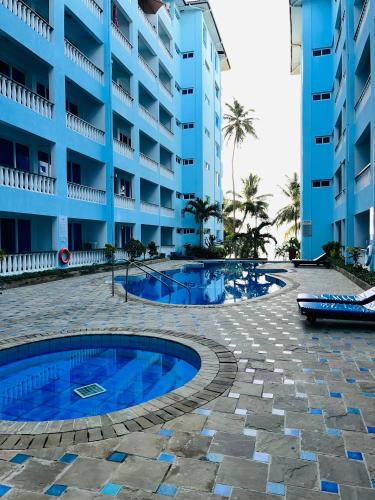The image depicts a narrow, outdoor pool area at a beach resort hotel, nestled between two buildings of the same establishment. Each building stands approximately seven stories high and is painted light blue with white railings. The overcast sky above lends a muted brightness to the scene, with white clouds obscuring the sun. At the far end of the courtyard, tall palm trees provide a tropical vibe.

Central to the image is an inviting pool with a free-form, kidney-shaped design, featuring many gentle curves and clad in cobalt blue tiles. Adjacent to this is a circular water feature, likely a hot tub or possibly a wading pool for children, similarly set into the stone decking. The stone paving around the pools is primarily gray with cobalt blue square accents adding a touch of elegance. Near the edge of the pool area, two lounge chairs are positioned between the pool and the hot tub, suggesting a perfect spot for relaxation. The water in both pools is vividly blue, creating a refreshing contrast against the neutral tones of the paving and the soft colors of the buildings.